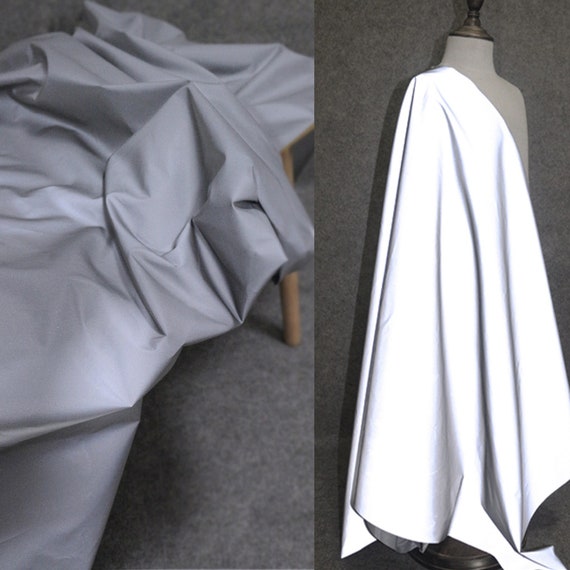This composite image consists of two vertically aligned rectangular photographs set side by side against gray carpet-like backgrounds. 

On the left, a piece of gray, crumpled fabric, resembling a man's dress shirt, rests on a light wooden structure, likely a table or stool, with its round legs visible. The fabric has a glossy texture, with folds and creases creating intricate patterns as it drapes over the wooden surface and extends onto the carpet, which has the look and texture of felt.

On the right is a headless and armless mannequin, similar to a seamstress figure, standing against a slightly darker gray backdrop. The mannequin features a bronze spindle top above the neck and a bronze base. Draped over one shoulder of the mannequin is a bright white cloth that reaches the ground, pleated vertically with dark gray creases and shadows enhancing its texture and form.